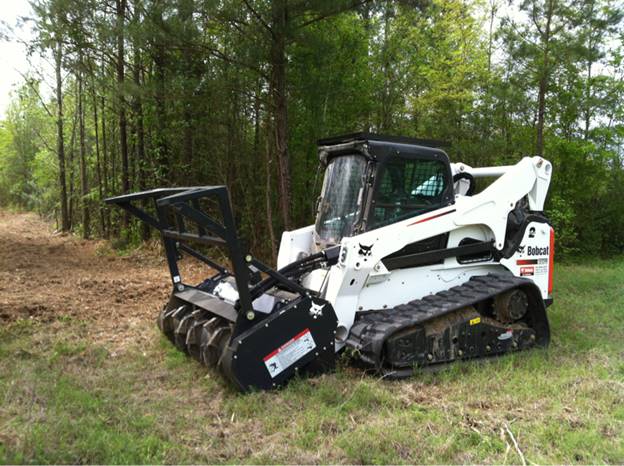In this detailed color photograph, a Bobcat branded tractor is prominently featured in a dense forest with a mix of green and dead brown grass under a light blue sky. The scene is bisected by a dirt pathway lined with dry leaves on the left. The Bobcat tractor, positioned slightly right of center, is predominantly white with black accents, including the cabin, safety-netted windows, and tracks. Red warning signs and the Bobcat logo with black lettering on a white background with a red border are noticeable. The tractor, which appears unmanned, is equipped with a front attachment featuring two large prongs and rototill blades, seemingly designed for heavy-duty tasks such as wood chipping or excavation. Tall, lush green trees surround the area, casting shadows over the scene and lending a sense of quiet seclusion to this rural, work-in-progress landscape.